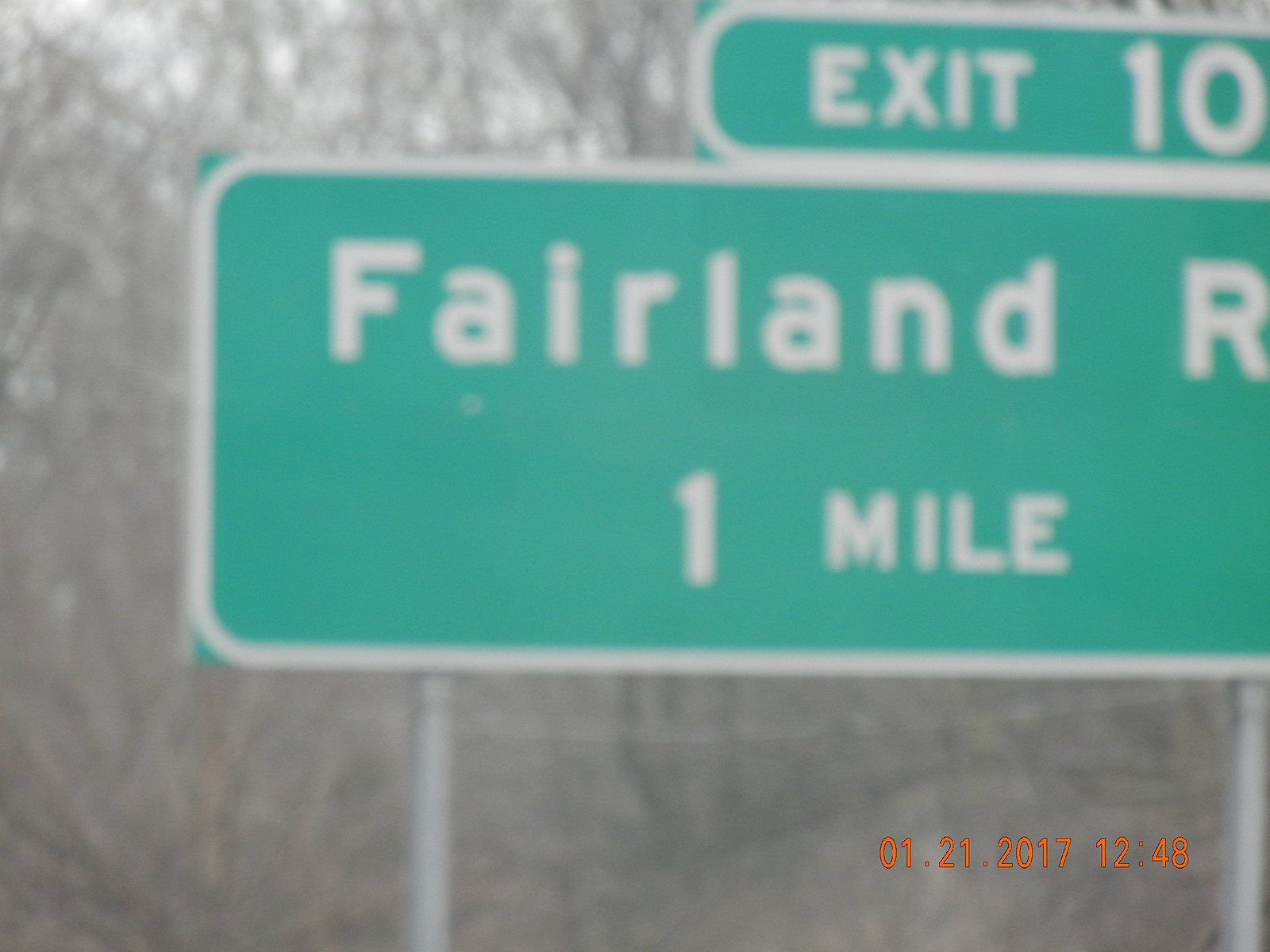The image depicts a highly blurry outdoor scene, obscuring many of the finer details. Dominating the photograph is a green rectangular street sign, mounted on metal poles, displaying in white text: "Exit 10" at the top, "Fairland R" in the middle, with the remainder of the word cut off, and "1 mile" at the bottom. A distinctive white border frames the sign. The background is filled with leafless trees, indicating a winter setting. In the bottom right corner, the image features an orange date stamp that reads "01.21.2017.1248," clearly superimposed on the photograph.